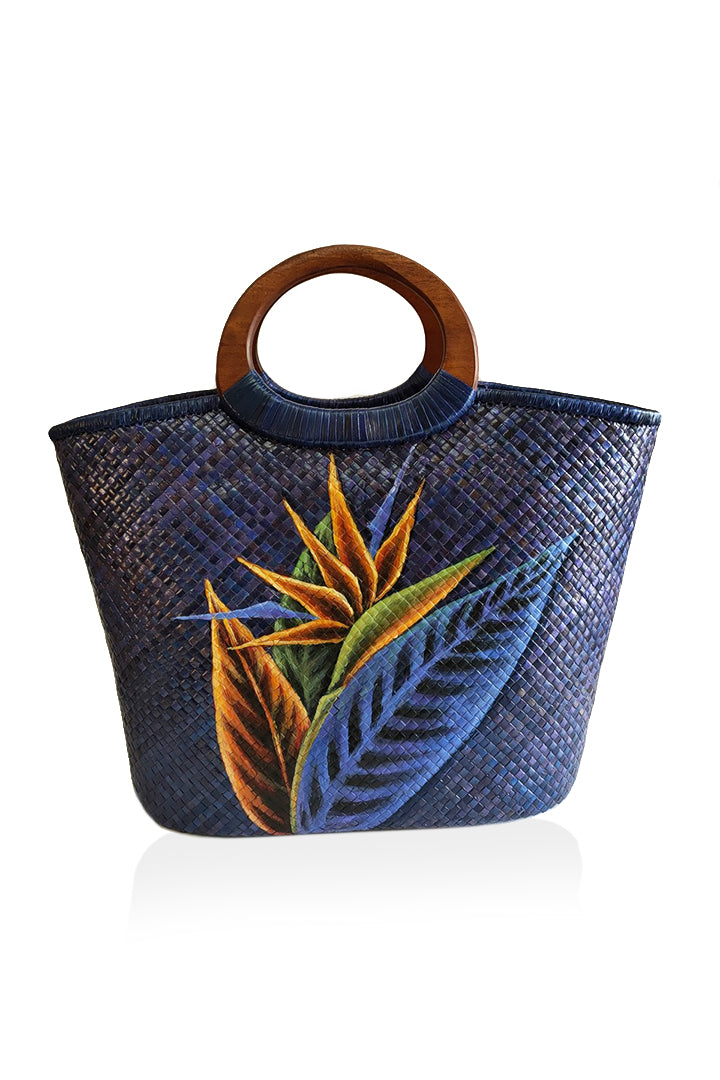This photograph depicts a medium-sized handbag crafted from intricately woven materials that blend various hues, including dark blue, purple, and black. The handbag features distinctive circular, oval-shaped wooden handles that are securely attached by looping thick thread multiple times, enhancing its artisanal appeal. The woven pattern forms a series of diamond-shaped squares, where the colors crisscross to create an eye-catching design. Centrally displayed on the front of the handbag is an elaborate illustration of a Bird of Paradise plant. The plant motif includes several leaves in vibrant shades: a bright blue leaf, an orangish-brown leaf, and a green leaf. Surrounding these are five larger, pointed fronds, with two smaller bright blue fronds positioned behind them. The texture near the handles transitions into a leathery dark blue, adding to the handbag's refined aesthetic.